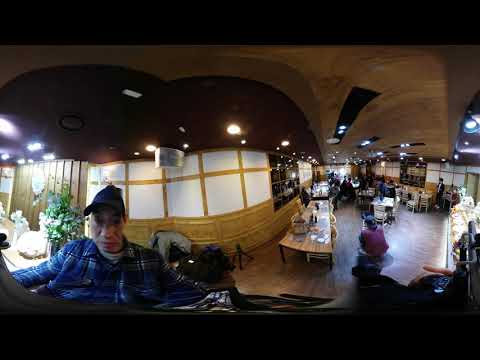This photograph, seemingly captured inside a restaurant or deli, is taken with a camera that distorts the image, giving it a fisheye effect. The setting features a wooden, brown-colored floor and a matching ceiling adorned with various lights and golden designs interspersed with white squares or windows. Prominently placed, an older man wearing a blue cap and a blue checkered shirt is seen not looking directly at the camera. 

To the right of the image, many people are seated at tables, with some standing. Several tables and chairs are visible throughout the scene, indicating a bustling atmosphere. There appears to be a small counter on the right side, potentially housing cakes, but it's somewhat ambiguous due to the image's distortion. Additionally, the top and bottom of the image are bordered by two horizontal black strips, framing the overall curved visual. Overall, while the distortion alters the exact proportions and shapes of the objects and people, the photograph clearly captures the lively, detailed interior of a dining establishment.